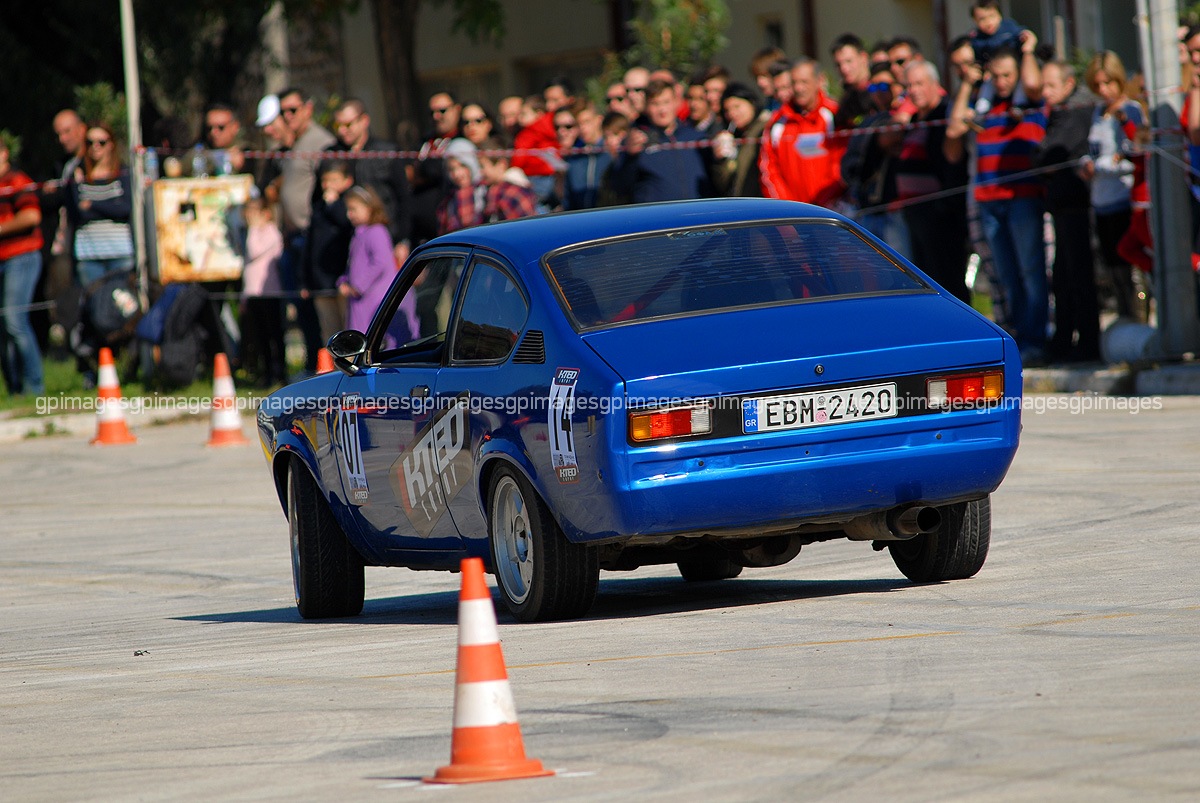The image captures the thrilling moment of a vintage rally race, focusing on a royal blue, two-door hatchback with distinct markings. The number "07" paired with "KTED export" emblazons the side, while the rear displays "14" and a white license plate reading "EBM 2420." The car, positioned in the center of the image, appears to be in motion with its wheels turned. Surrounding the scene, a crowd of spectators, including some children, stands on the sidewalk behind two thin ropes for safety. They watch attentively from a grassy area as the car navigates around several orange parking cones set across the course. White text reading "EBM2420" is visible on the license plate, indicating its United Nations affiliation. The overall atmosphere exudes excitement as onlookers witness this dynamic auto event.